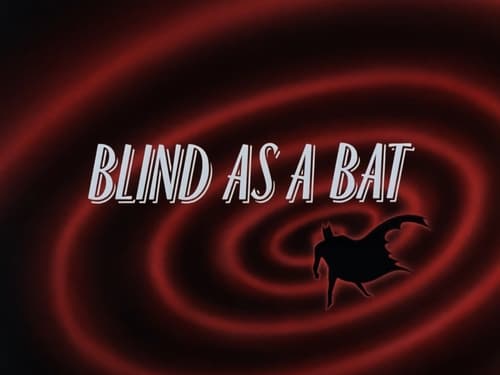The image features a stark contrast of black, white, and red to create a striking visual effect. Dominating the scene is a black background, overlaid with concentric red swirls that appear like ripples expanding from a central point. These red swirls are slightly muted and out of focus, adding depth and motion to the composition. In the middle, bold white capital letters proclaim "BLIND AS A BAT," with a subtle 3D effect that lends the text extra dimension. Positioned directly below the word "BAT" is the black silhouette of a bat, or possibly a figure reminiscent of Batman, with a swirling cape that extends to the right, resembling a flag caught in the wind. The overall impression is a compelling graphic with an intense, almost hypnotic atmosphere.